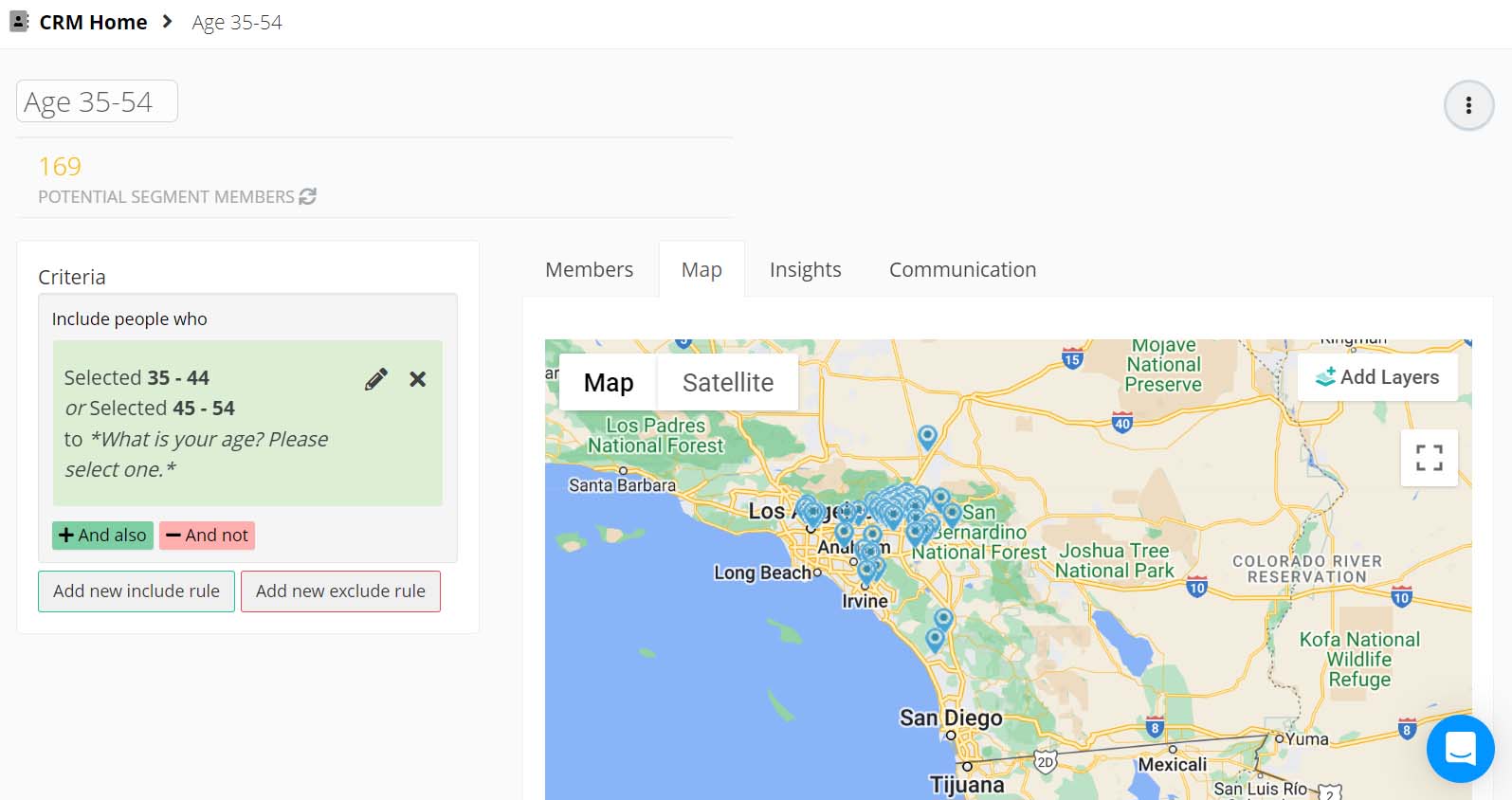The image appears to be a detailed map of California, prominently displaying various geographic and administrative features. The map highlights cities such as San Diego and Los Angeles, with blue icons densely clustered above Los Angeles. The Pacific Ocean is visible on the left side of the map, with notable coastal locations such as Long Beach and Santa Barbara clearly marked. The map also shows significant natural areas, including the Los Padres National Forest in the top left, Joshua Tree National Park, San Bernardino National Forest, and Kofa National Wildlife Refuge.

Yellow lines crisscross the map, alongside beige landmasses and green areas indicating different regions or zones. In the upper part of the map interface, there are several tabs labeled "Map," "Members," "Insights," and "Communication," with "Map" being actively highlighted.

On the top left of the image, there is a demographic segment description stating "Ages 35 to 54" with "169 potential segment members." Criteria are listed, including groups of people aged between 35 to 44 and 45 to 54, as indicated by a green-highlighted area. The prompt "To what is your age?" invites selection, with accompanying green "+" and red "-" buttons for adding or subtracting age ranges. Additionally, there are options to "Add new include rule" in green and "Add new exclude rule" in red, allowing for further customization of the segment criteria.